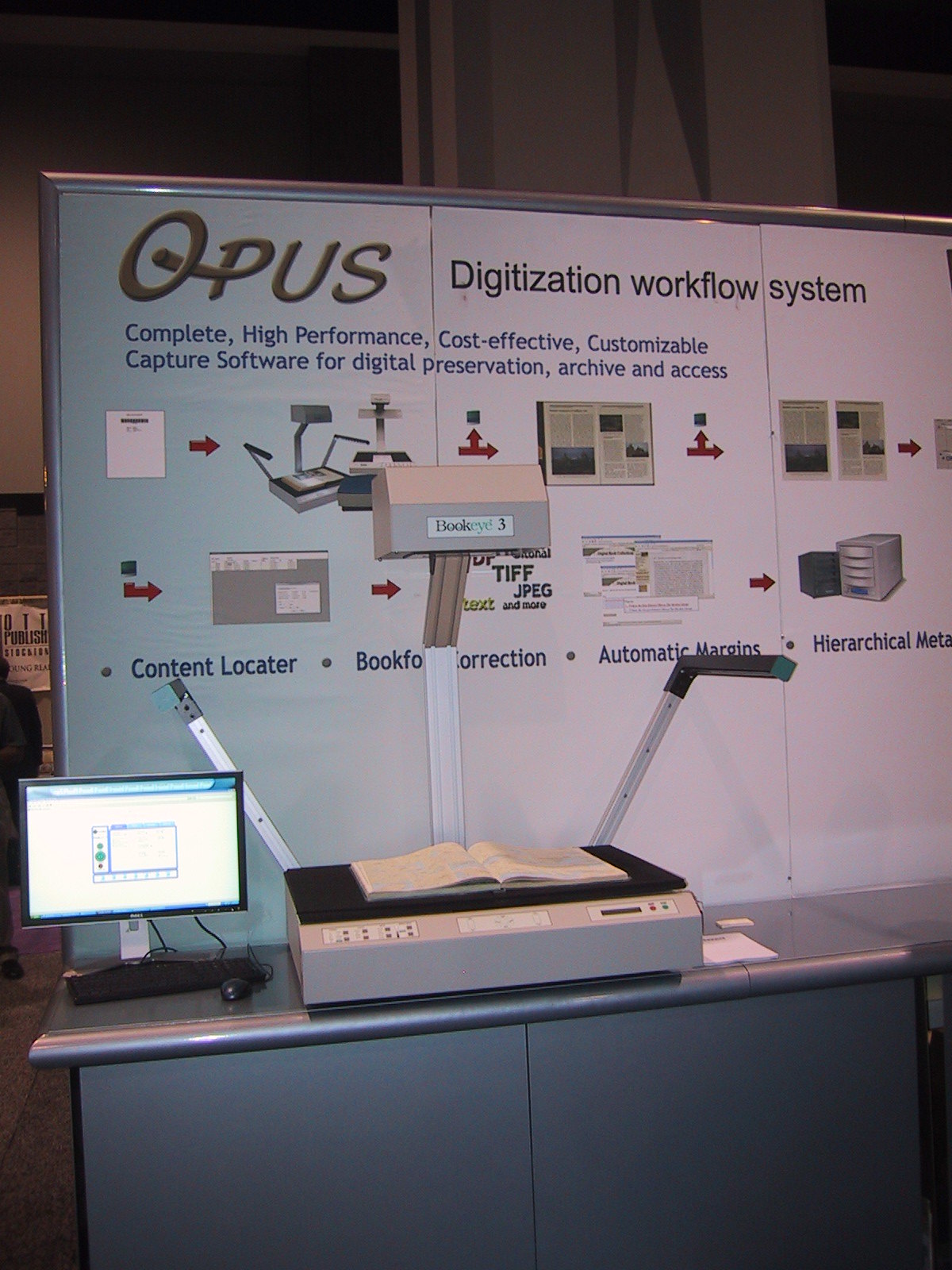The image showcases a detailed setup for a digital preservation and archiving workflow system. In the center, there is a large whiteboard with black writing and images, prominently displaying the title "Opus Digitization Workflow System." This system is described as a "complete high-performance, cost-effective, customizable capture software for digital preservation, archive, and access." Several photos and arrows are arranged on the board, with additional readable text such as "Contact Locator" and "Automatic Margins." Some letters on the board are partially obscured by a machine.

On the table in front of the board, there is a small computer monitor on the left, accompanied by a computer mouse. To the right of the monitor, a scanner or possibly an overhead projector with a book laid open on it occupies the central part of the table. This machine seems to serve as the primary equipment for the digitization process being promoted on the board. The arrangement suggests a professional or educational setting, perhaps a classroom, where digital archiving and preservation techniques are being exhibited or taught.